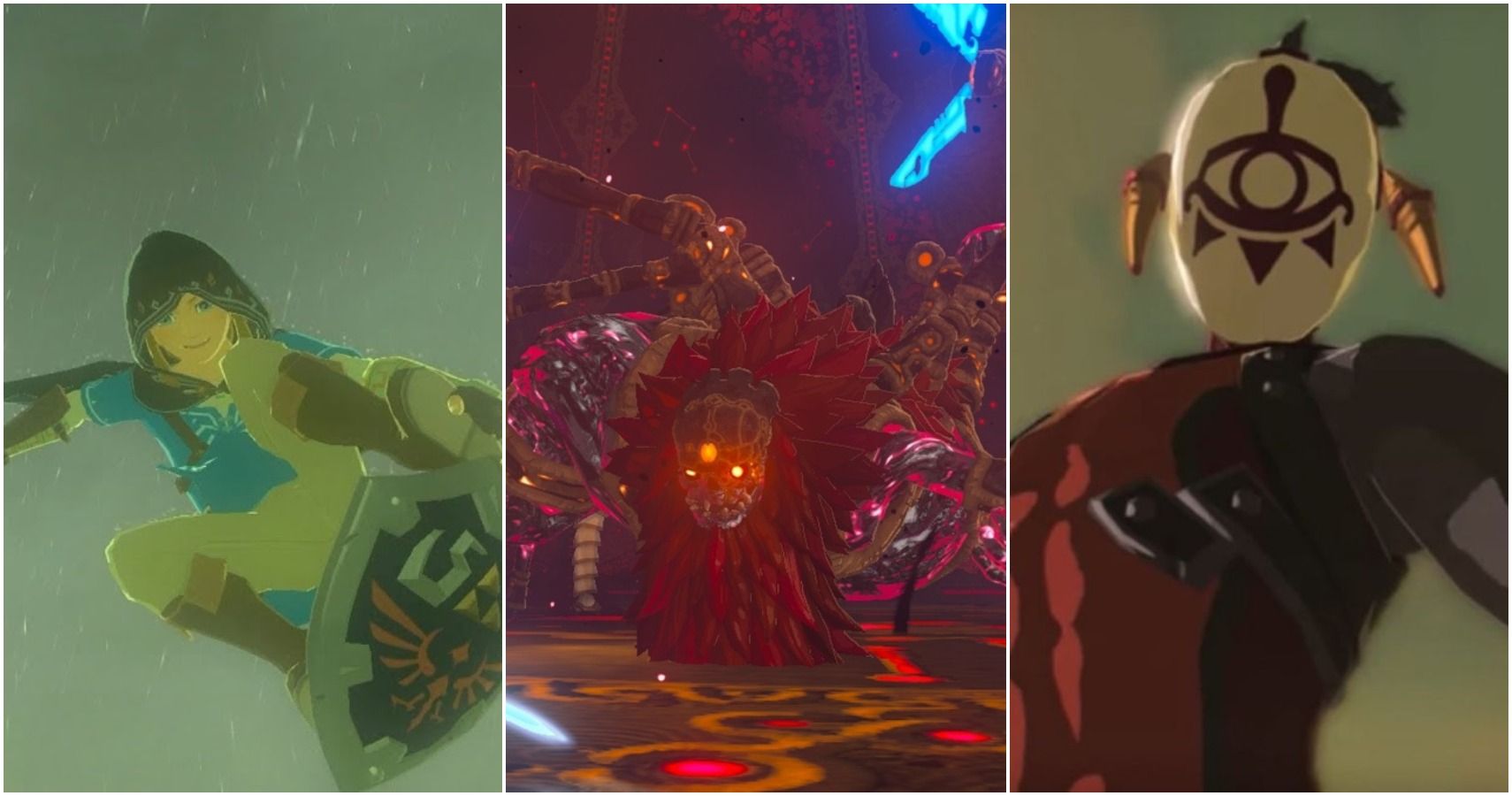This image is a three-panel digital artwork, each panel illustrating distinct, dynamic characters rendered with vibrant colors and intricate details. 

In the left panel, a young person, possibly a female, is depicted in motion, gliding through the air using a shield as a makeshift snowboard. She is dressed in a blue top, green pants, and knee-high green boots, with raindrops suggested in the scene, adding a sense of action and movement. 

The middle panel features a menacing creature with a red-feathered mane and numerous tentacles. The creature's face resembles a mask with glowing orange eyes, set against a dark and eerie background, possibly indicating an indoor or shadowy environment. 

The right panel showcases a muscular man wearing a striking white mask emblazoned with a single, large eye. The mask obscures his facial features completely, and he has horns protruding from either side of his head. He is attired in a red shirt, standing firmly with an enigmatic and intimidating presence. 

Each panel is distinct yet unified under the shared theme of human-like characters, blending elements of fantasy and intensity.